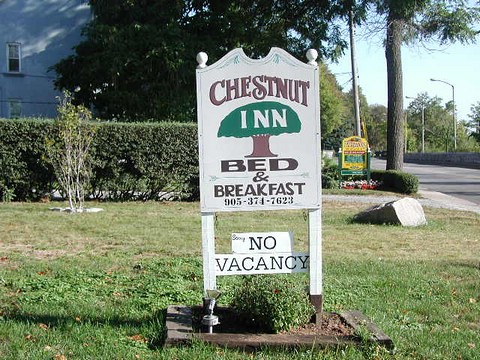The photograph captures a charming, white wooden sign for the "Chestnut Inn Bed and Breakfast," prominently featured in a lush, green lawn. The top part of the sign reads "Chestnut" in brown text, accompanied by a logo of a green treetop with a brown trunk and the word "Inn" written across it. Below this, in smaller text, is the contact number "905-374-7623." Beneath this primary sign, there's a secondary white sign stating "Sorry, No Vacancy" in black serif font. Anchoring the sign to the ground are sturdy white posts set into a cement base, surrounded by green grass and scattered shrubs.

In the background, partly obscured by foliage, is a light blue building. Large trees, including one prominently in the top right corner and another along a nearby street, frame the setting. Adjacent to the street and blending into the scene, there's a yellow sign that appears to denote a farmer's market, though its details are indistinct. The atmosphere captures a tranquil, welcoming rural or suburban environment, invoking the cozy appeal of a bed and breakfast.